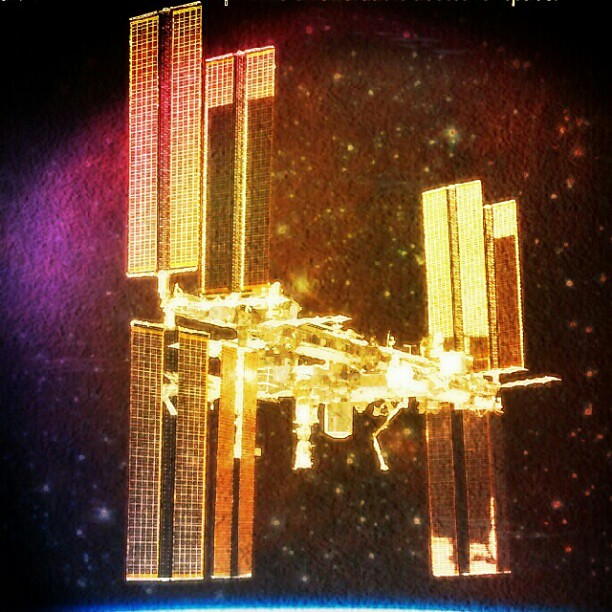The image showcases a detailed scene of a space station, potentially the International Space Station or a similar space vehicle, positioned centrally in the vastness of outer space. The space station appears slightly tilted to the right, viewed from a flat diagonal perspective. It is adorned with solar panel wings on the left and right, extending vertically upward and downward, capturing a golden hue from the sun's rays, possibly shining on it after emerging from darkness. 

Surrounding the space station, the background is a star-studded expanse, with numerous small, white stars that also seem to reflect a golden light. To the left of the station, a distinct purplish haze creates a soft contrast. Observers note a potential planet or moon in the backdrop, adding to the depth and wonder of the scene. The space station itself is a complex structure, featuring eight solar panels total—four on each side—along with various metallic components that intricately connect the central body. The overall image combines golden highlights on the station, a purple hue on the left, and intermittent black shading on the panels, crafting a visually striking representation of space exploration.